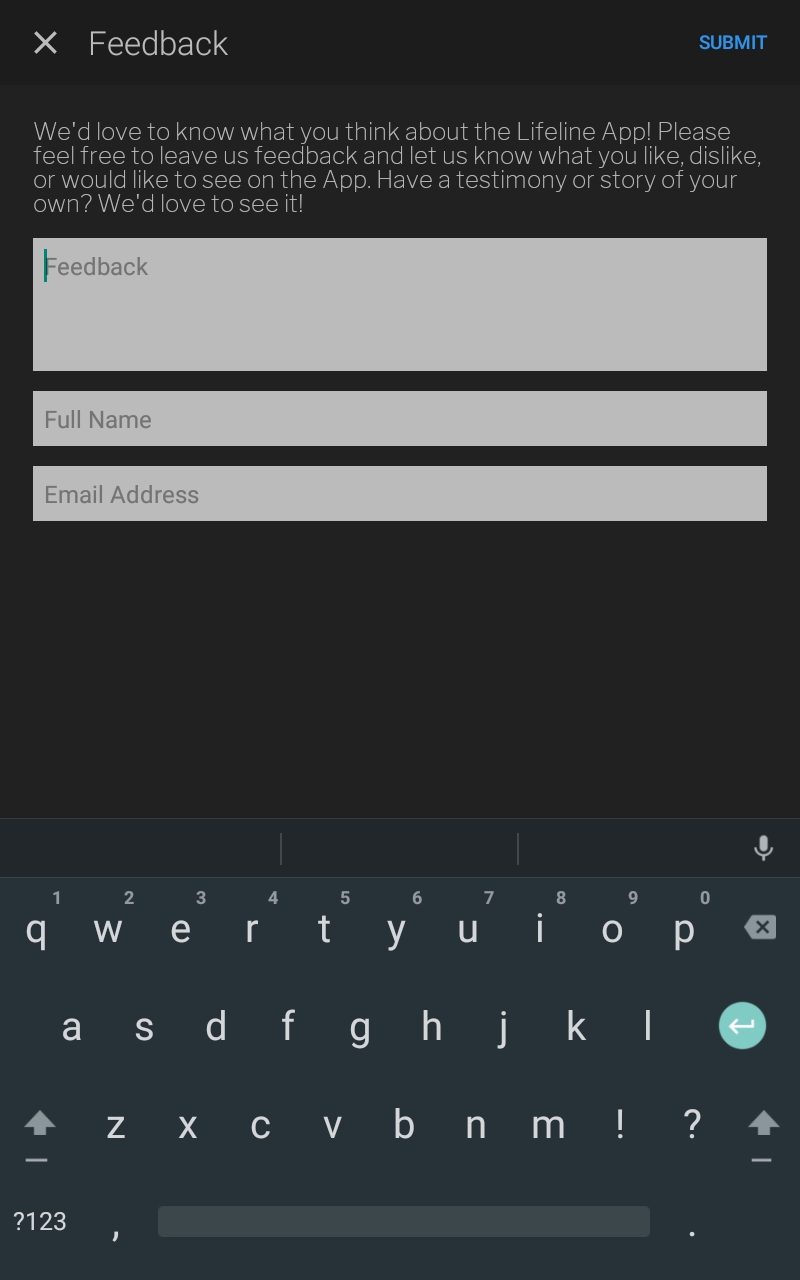In this image, the upper portion features a black background, while the lower portion transitions to a slightly dark grey shade. Dominating the lower part is a QWERTY keyboard, showcasing characters in high relief. In the upper left corner, the white text "FEEDBACK" is prominently displayed. Adjacent to this on the left, a close button marked by an "X" is visible. On the upper right corner, a blue "SUBMIT" button catches the eye.

Below the "FEEDBACK" heading on the left, the text reads: "We'd love to know what you think about the Lifeline app. Please feel free to leave us FEEDBACK and let us know what you like, dislike, or would like to see on the app. Have a testimony or story of your own? We'd love to see it."

Further down, there are fields for user input: one labeled "FEEDBACK" for users to enter their comments, another labeled "Full Name" for the user's name, and a final space labeled "Email Address" for their email. This image represents the FEEDBACK submission form of the OnAir Lifeline app, inviting users to share their thoughts, testimonies, or stories, and to leave their full name and email address to receive a response.